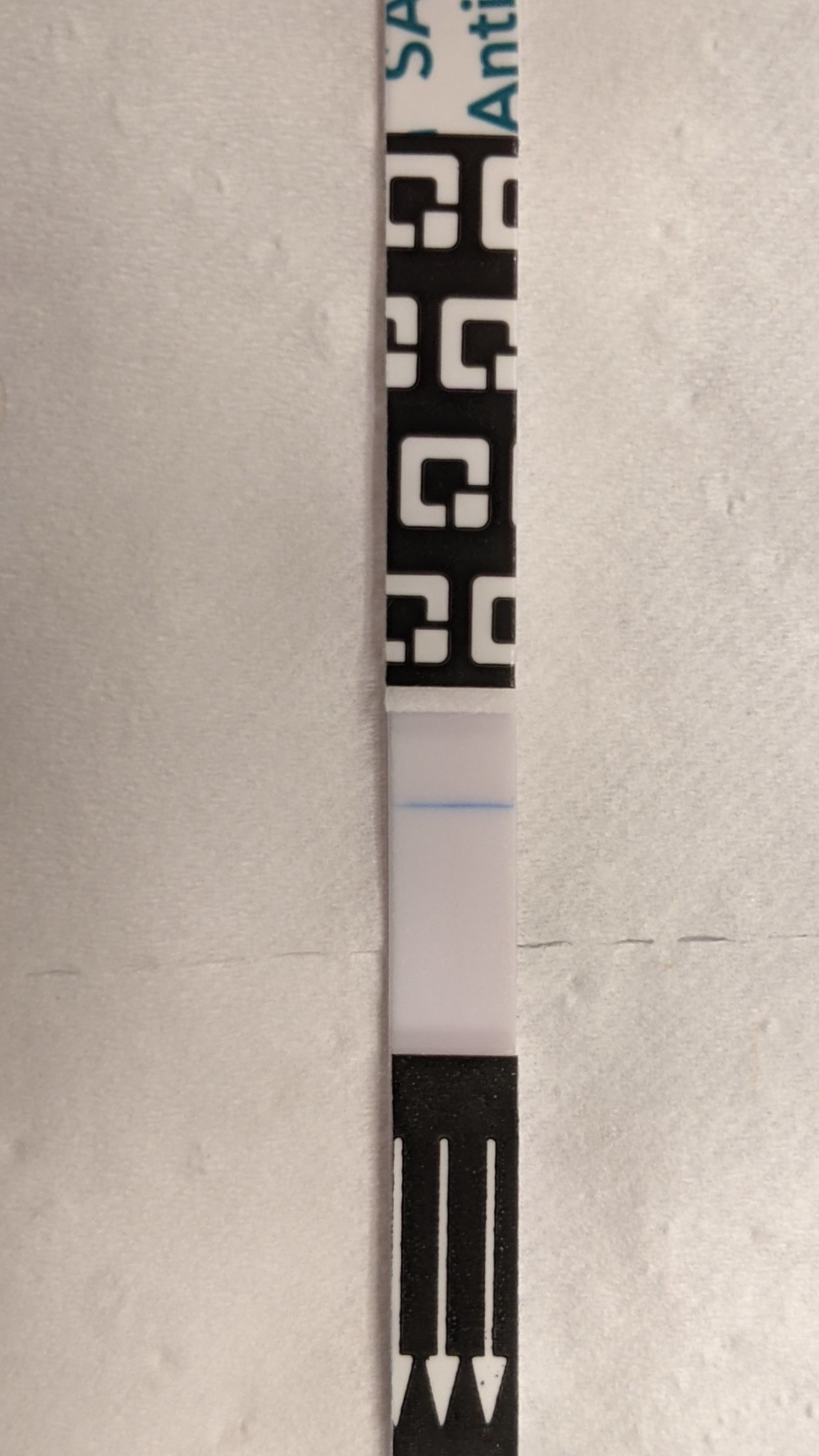The image depicts a testing device that resembles either a COVID-19 test or a pregnancy test, resting on two connected pieces of toilet paper. The toilet paper has a serrated line running horizontally across the background, approximately halfway down the picture. The upper part of the test is white and features green lettering partially spelling out "SA" and "ANTI," with the rest of the letters cut off. Below this, a black section adorned with white designs—resembling small squares with their bottom right corners separated—is visible. 

The test segment itself has a white area displaying a single blue line, indicating the result. At the bottom, another black section features three white arrows pointing downward toward the base of the stick, suggesting it is a dipstick-type device. The toilet paper in the image has small dents at its top, possibly from being handled while being torn from the roll.